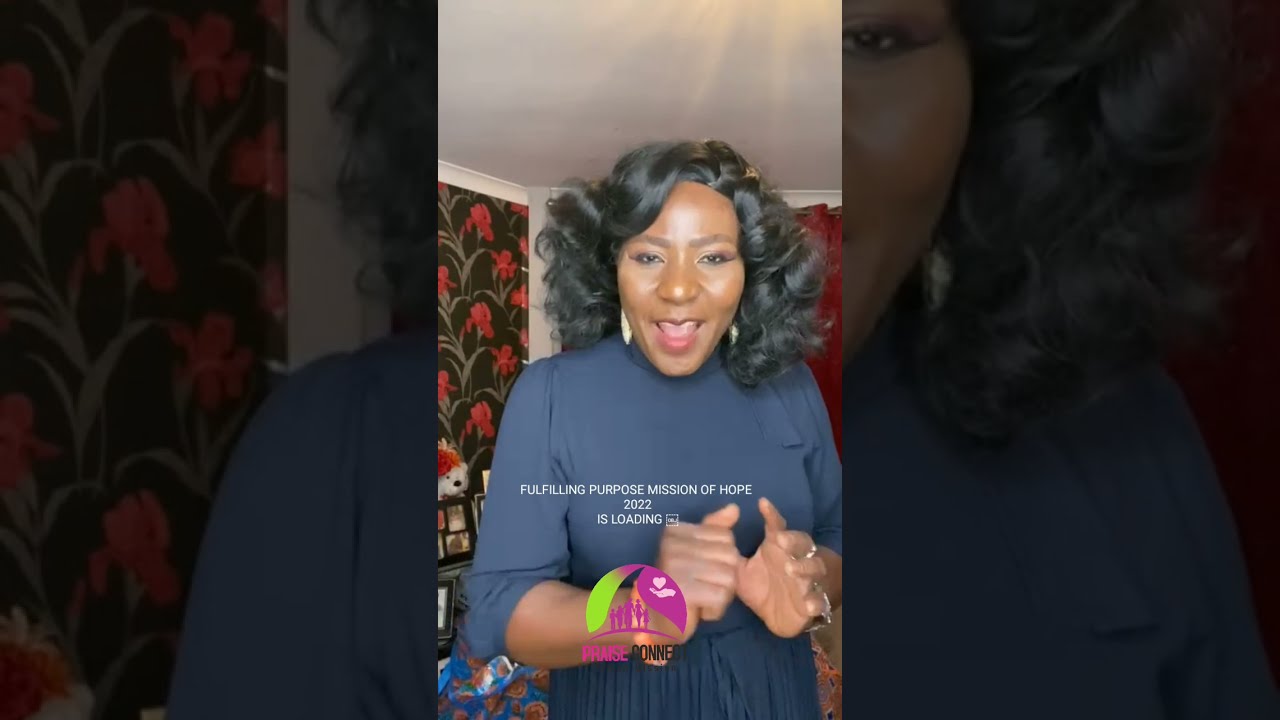The photograph is a visually intriguing composition showcasing a black woman with vibrant, curly black hair, dressed in a blue dress that resembles a turtleneck blouse with puffy sleeves ending near her elbows. The image is segmented into three horizontal sections: the left and right sections are darker and slightly grayed out, showcasing the sides of the woman's face and torso, while the middle section exhibits the full, clear image of her facing forward. Her mouth is open as if she's speaking, and her hands are held out in front of her, possibly gesturing.

In the middle image, she is surrounded by a room adorned with dark wallpaper featuring red flowers, along with a red curtain and a visible ceiling light glare. There is some white text across her chest area that is too small to read clearly, along with a purple and green emblem near her right hand depicting small figures walking over a horizon with more unreadable text beneath it. The caption on the image reads, "fulfilling purpose mission of hope 2022 is loading." The darkened borders on the left and right sections provide a striking contrast, framing the central, more illuminated and detailed depiction of the woman.